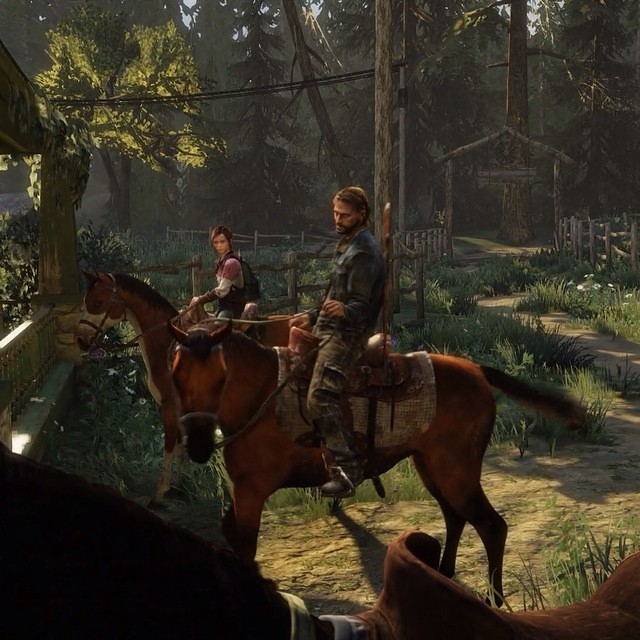In this detailed image, a screenshot from the video game The Last of Us exclusively for PlayStation, we see two characters, Ellie and Tommy, on horseback. Set during a sunny day, the scene unfolds in a lush, forest-like, possibly a ranch area. Ellie, a young girl with dark brown hair, dons a light purple, white, and dark purple sweatshirt, and carries a backpack. She rides a pinto horse with a distinctive black mane, white stockings, and a star marking on its face. Alongside her is Tommy, who resembles actor Viggo Mortensen. He has stubble, dark blonde hair, and appears to be in his mid-30s. Tommy is dressed in a dirty denim button-up shirt, camouflage pants, and army-style boots, and sits astride a brown horse with a black muzzle, mane, and tail, equipped with an English saddle and a full bridle. The foreground features Tommy's horse's mane and pommel, and he carries a rifle slung over his back. The background showcases large trees, a wooden fence made of logs, a pathway, a wagon wheel entryway, and power lines, enhancing the rustic, pastoral setting.